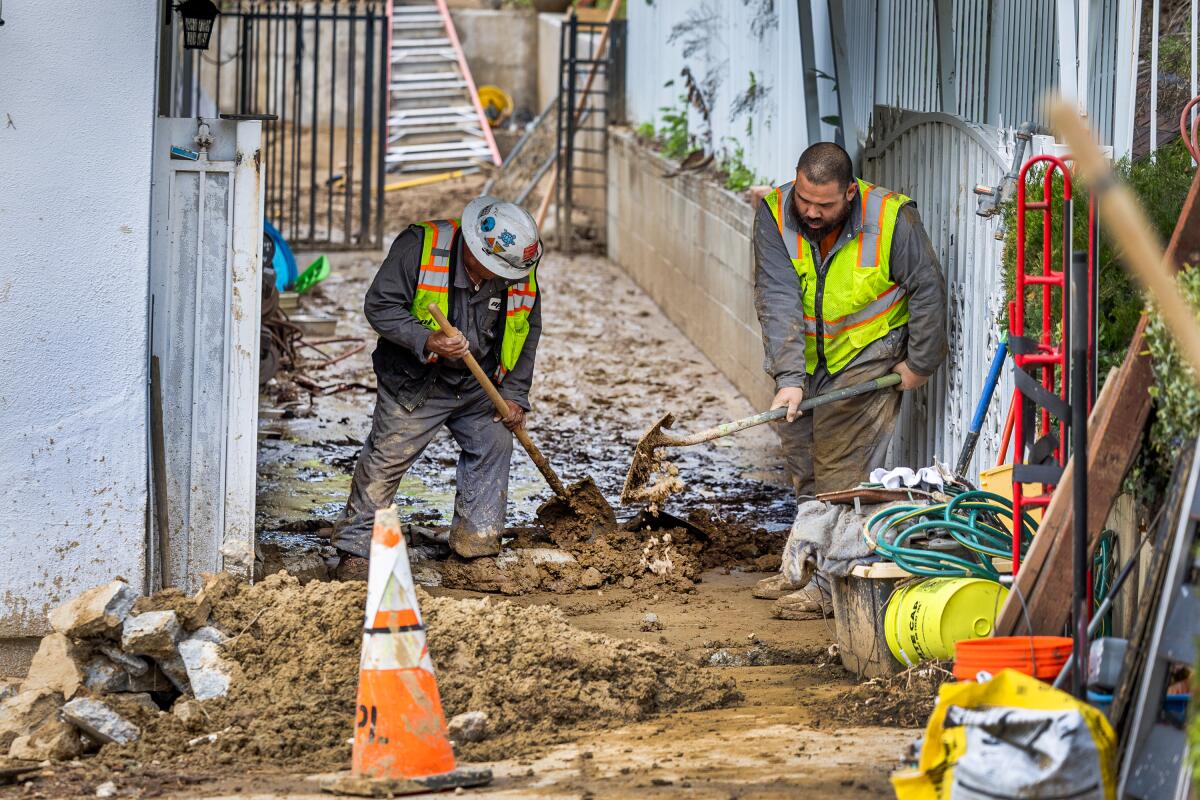This color photograph captures a scene of two construction workers laboring in a muddy alleyway between two buildings, likely cleaned after a flood. The alleyway is cluttered with wet dirt, mud, and broken rock. The worker on the left is donned in brown pants, a gray jacket, a high-visibility green vest, and a white hard hat adorned with stickers. Next to him, the second worker is wearing blue jeans, a gray jacket, and a similar green high-vis vest. Both men are actively engaged in the task: one wielding a shovel and the other using a tool that appears to be a pickaxe-like device. The alley is framed by a white gate on the right, which stands open behind the workers. Other notable items in the scene include a hand truck, a couple of five-gallon buckets, a wrapped-up hose, and an orange caution cone situated in front of the workers. Additionally, two ladders can be seen, one towards the back and one to the side of the image. The environment is heavily mud-splattered, underlining the heavy, dirty work the men are undertaking.